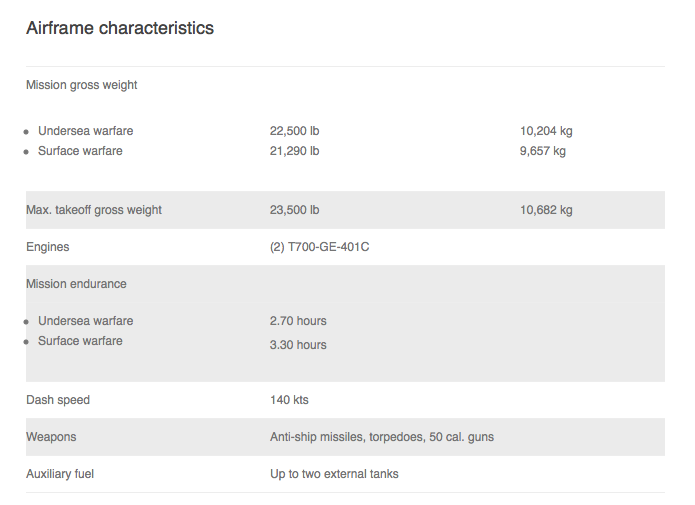The image is an Airframe Characteristics Chart for Nature Rove, prominently featuring "Airframe Characteristics" in bold at the top. It details various specifications and configurations. The chart lists "Mission Gross Weight" with two bullet points: "Undersea Warfare" at 22,500 pounds (10,204 kilograms), and "Surface Warfare" at 21,290 pounds (9,657 kilograms). The "Max Takeoff Gross Weight" is noted as 23,500 pounds (10,682 kilograms). It specifies the engines as two T-700 GE-401C models. The "Mission Endurance" is detailed with "Undersea Warfare" at 2.7 hours and "Surface Warfare" at 3.3 hours. The "Dash Speed" is identified as 140 knots. Weapons systems include anti-ship missiles, torpedoes, and .50 caliber guns. Additionally, the aircraft can carry up to two external auxiliary fuel tanks.